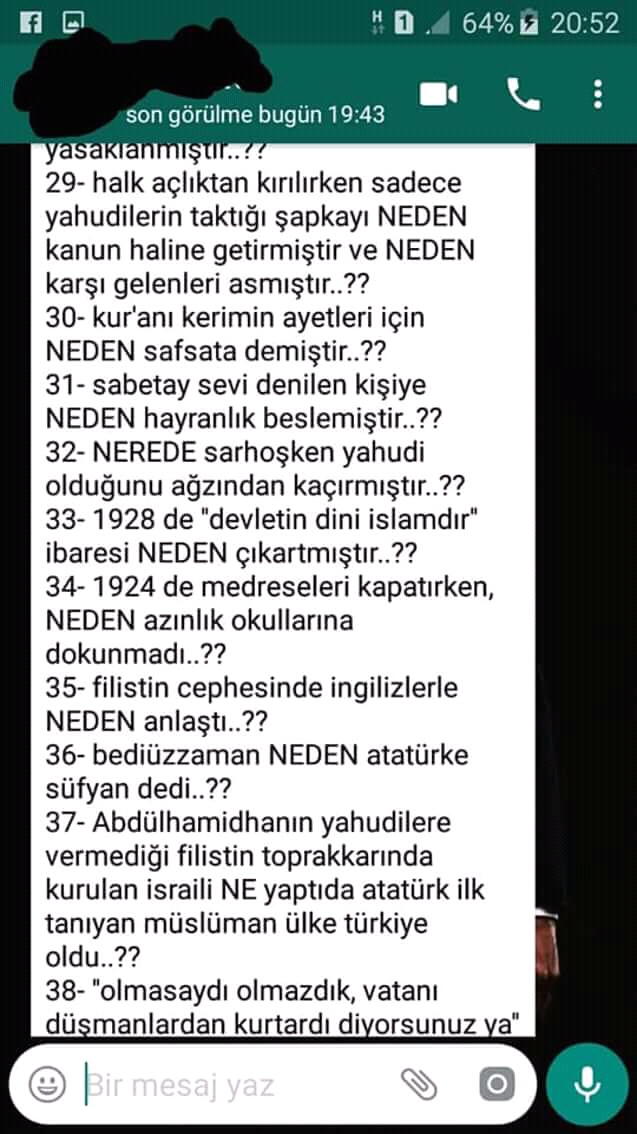This is a detailed screenshot of a messaging app on an Android phone, displaying a text message written in an unfamiliar language that might be Turkish. The interface of the app features a green and black color scheme. The status bar indicates that the phone has one sim card installed, poor cell service, and 64% battery remaining. It is currently 8:52 PM (20:52). The screenshot captures a long text message with black text, showing item numbers 29 to 38. There are also visual elements such as a percentage in the corner and a FaceTime option, indicating that it's a screen capture from the user's device. Numbers are interspersed within the text, suggesting a list format.